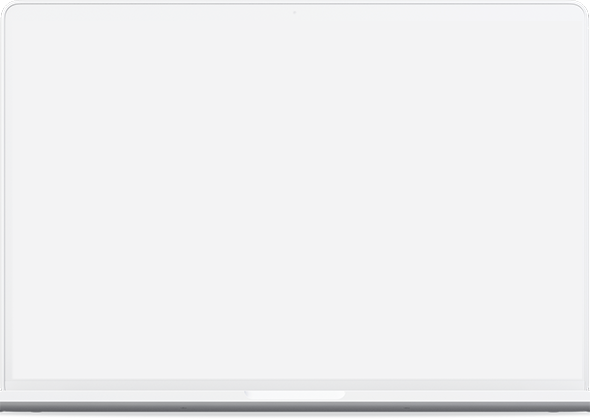This image features a screenshot of a blank page displayed in a rectangular format. The page is marginally wider than it is tall. The primary color of the page is a light purple, with a consistent hue throughout, except for a narrow border of darker purple extending along the left margin and across the top. The page's top corners are rounded, adding a subtle softness to its silhouette.

Beneath the top edge, a light gray stripe spans horizontally from the left to the right. This stripe is slightly wider than the darker purple border at the top. Below this, there is a narrower band of a lighter gray, also running horizontally from the left side to the right side. Directly below this lighter gray band, a very thin, dark line extends across the width of the page. This dark line is approximately an eighth of an inch wide. Beneath it lies another very thin strip of light gray, completing the series of horizontal lines.

The lower two corners of the page are squared off, providing a sharp contrast to the rounded top corners. The overall design is simple and uncluttered, with no text or images breaking the expanse of blank space.